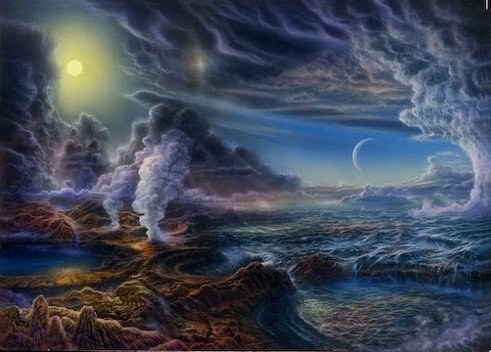The painting depicts a surreal and expansive landscape set on what appears to be an extraterrestrial planet, far removed from our solar system. Dominating the top left corner of the image, a radiant yellow sun casts its light upon the scene, surrounded by an array of clouds. In contrast, the top right corner features a substantial black cloud from which a menacing water spout or tornado emerges, churning a vast, turbulent blue body of water that stretches from the center down to the bottom right corner, culminating in a round whirlpool near the land.

The terrestrial expanse itself is a rugged terrain, cloaked in smoky vapors and riddled with steam vents. The rocky surface is predominantly brown and scattered with various rock formations and molten areas. Amidst this alien landscape, multiple round pools of water punctuate the ground, further enhancing the otherworldly atmosphere. There's also a faintly visible quarter moon to the right, adding another layer of mystique to the sky already populated with ominous dark gray and black clouds. This chaotic and captivating blend of elements creates a strikingly dramatic and fantastical landscape.